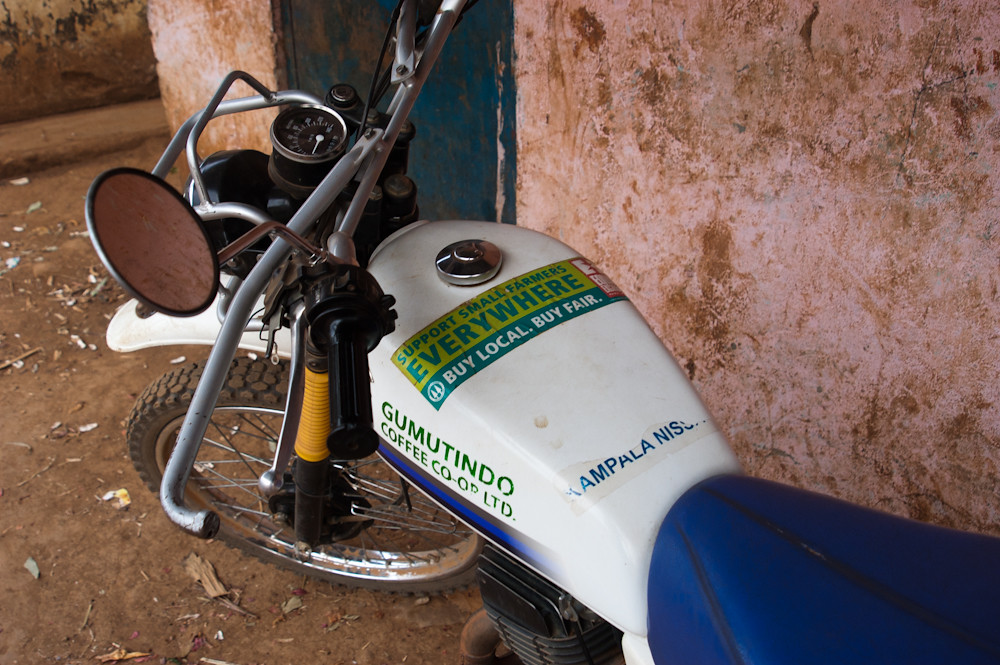In this close-up image, a beat-up, old-school motorcycle, leaning against a dilapidated, light pinkish wall stained with brown dirt, evokes a scene from a third-world country. The motorbike, characterized by its white body and blue seat, sits in a dirty outdoor area cluttered with debris and trash, especially on the left side. The ground is a dark, light-brown shade, further accentuating the gritty environment. Prominently displayed below the handlebars, a bumper sticker on a green background reads, "Support small farmers everywhere, buy local, buy fair," in blue and white fonts. Furthermore, the side of the engine carries the name, "Gumutindo Coffee Co-op Ltd." The wall behind features a partially visible green door, adding to the rustic and worn ambiance of the setting. One black handlebar and a single mirror, along with one visible wheel, complete the picture.